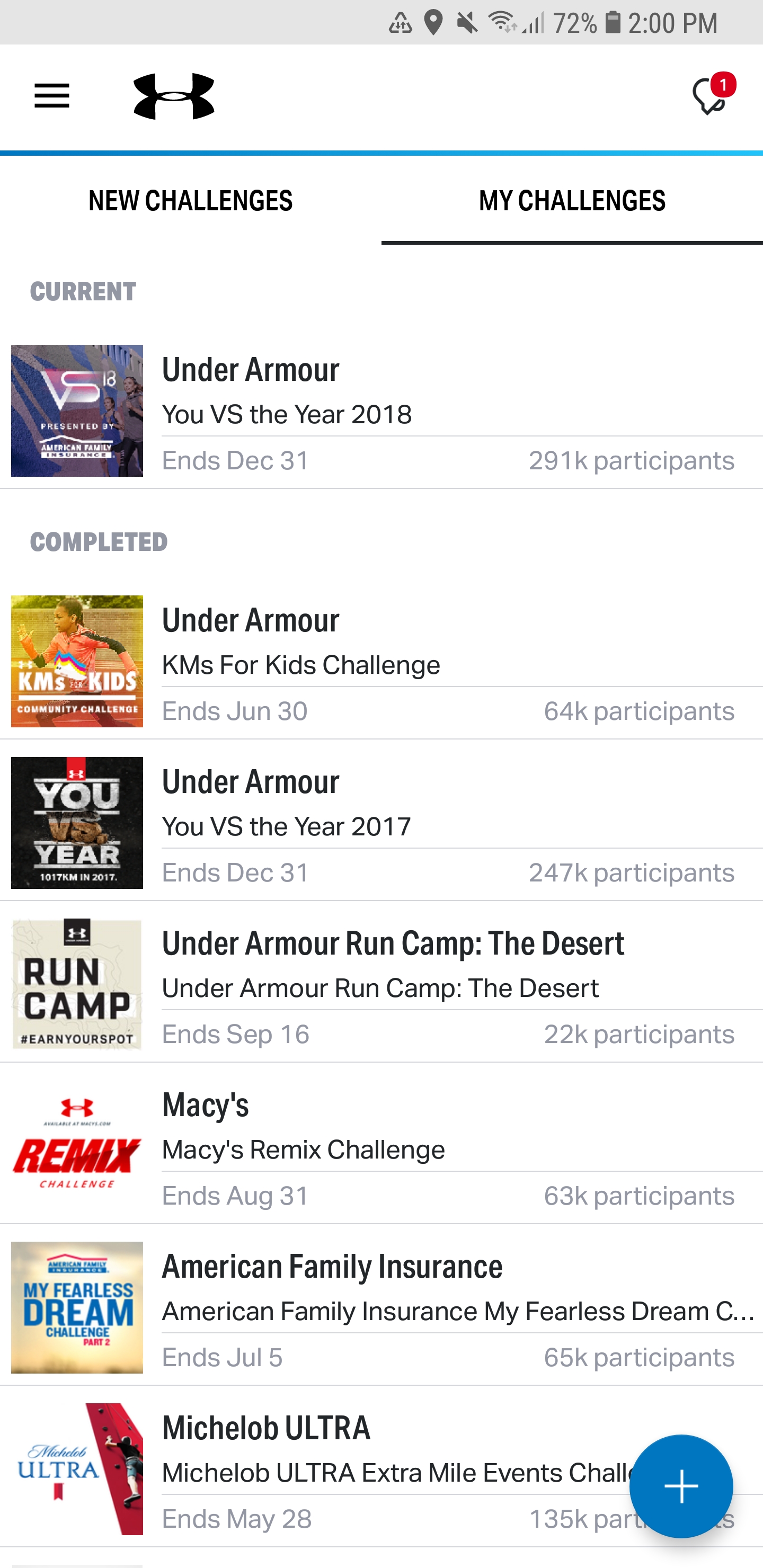This is a detailed screenshot of the Under Armour app displayed on an Android device. The familiar Under Armour logo is prominently visible, confirming the app's identity. The device status bar shows various icons: the standard Android icons for location access, muted volume, full Wi-Fi connectivity, nearly full cellular service bars, 72% battery life, and the device time set at 2 PM.

At the top-left corner of the screen, there is a menu icon, followed by the Under Armour logo next to it. On the top-right corner, there is an alert icon for location services. The app interface features two main tabs: "New Challenges" and "My Challenges," with the user currently viewing the "My Challenges" tab. 

Under the "My Challenges" section, the screen is divided into two subsections: "Current" and "Completed" challenges. Under "Current," a prominent challenge titled "Under Armour U vs the Year 2018" ends on December 31st, boasting participation from 291,000 individuals. 

The "Completed" challenges listed are:
1. "KMS for Kids Challenge" which ended on June 30th, with 64,000 participants.
2. "Under Armour U vs the Year 2017" which concluded on December 31st, with 247,000 participants.
3. "Under Armour Run Camp the Desert" which wrapped up on September 16th, attracting 22,000 participants.
4. "Macy's Remix Challenge" which ended on August 31st, with 63,000 participants.
5. "American Family Insurance by Fearless Dream" which concluded on July 5th, involving 65,000 participants.
6. "Michelob Ultra Extra Mile Events Challenge" which ended on May 28th, with 135,000 participants.

This detailed layout provides a structured view of both ongoing and past challenges, along with critical user engagement statistics for each.